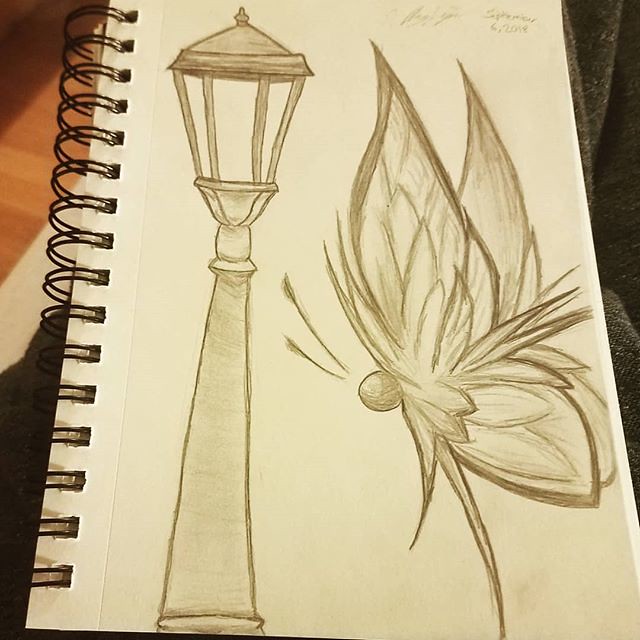This photograph showcases a page from a spiral-bound sketchbook, with the binding clearly visible on the left side. The pencil sketch on the page depicts an old-fashioned lamppost, reminiscent of those found in historic neighborhoods or city centers. Adding an element of whimsy, a mysterious creature with large, pointed, butterfly-like wings and a round, head-like shape can be seen on the left side of the lamppost. This fantastical figure, resembling a fairy but without human facial features, has a couple of elongated lines extending from its body and possesses delicate antennas sprouting from its head. The artist signed the piece at the top left of the page, although the signature is undecipherable. However, the date, "September 6th, 2018," is faintly visible. The notebook appears to be resting on a blanket or possibly the artist's lap, providing a cozy backdrop to the creative scene.